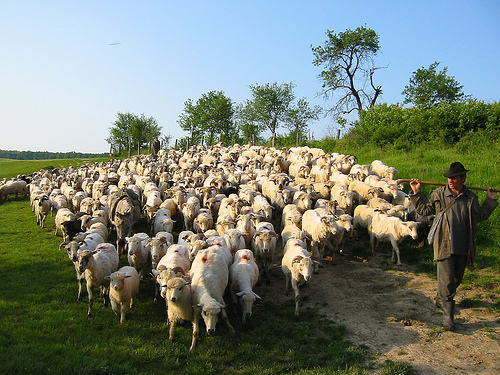In a picturesque countryside setting, this detailed color photograph captures a shepherd leading his closely packed herd of sheep down a dirt road. The shepherd, a white man, is depicted on the lower right side of the image. He wears a dark gray tunic shirt, dark pants, black boots, and a black hat. He carries a cane or walking stick propped on his shoulders behind his neck, with both arms bent at the elbows. Over his shoulder, he slings a gray crossover bag. The herd of sheep, possibly sheared, is densely grouped and spans almost the entire width of the image, narrowing slightly as they approach the bottom of the frame. The road they traverse is bordered by patches of green grass. In the background, a light blue sky stretches overhead, framed by a line of green trees on the horizon, interspersed with a small hill covered with grass and bushes. The image is captured from a slightly elevated vantage point, providing a comprehensive view of the scene that emphasizes the natural landscape and the harmonious pastoral activity.